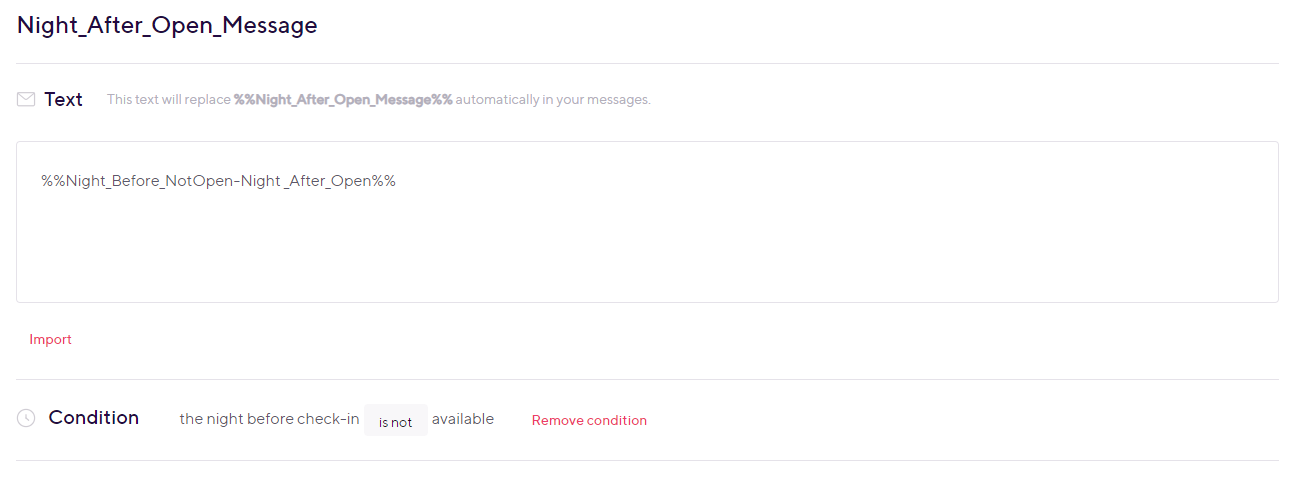The image depicts a user interface likely from a hotel management software. The visible text states:

"night_after_open_message text."

This placeholder text is intended to be automatically replaced in your messages with:

"%%night_before_not-open-night_after_open%%."

Each word in the text box begins with a capital letter. Below the text box is a red "Import" button, indicating that clicking it would import the specified message. 

Additionally, there's a "Condition" section which reads: "The night before check-in is not available." Adjacent to this is a red "Remove Condition" button, allowing the user to delete the specified condition. 

This interface appears to be part of a tool used by hotel managers or front desk staff to manage room availabilities and check-ins effectively.